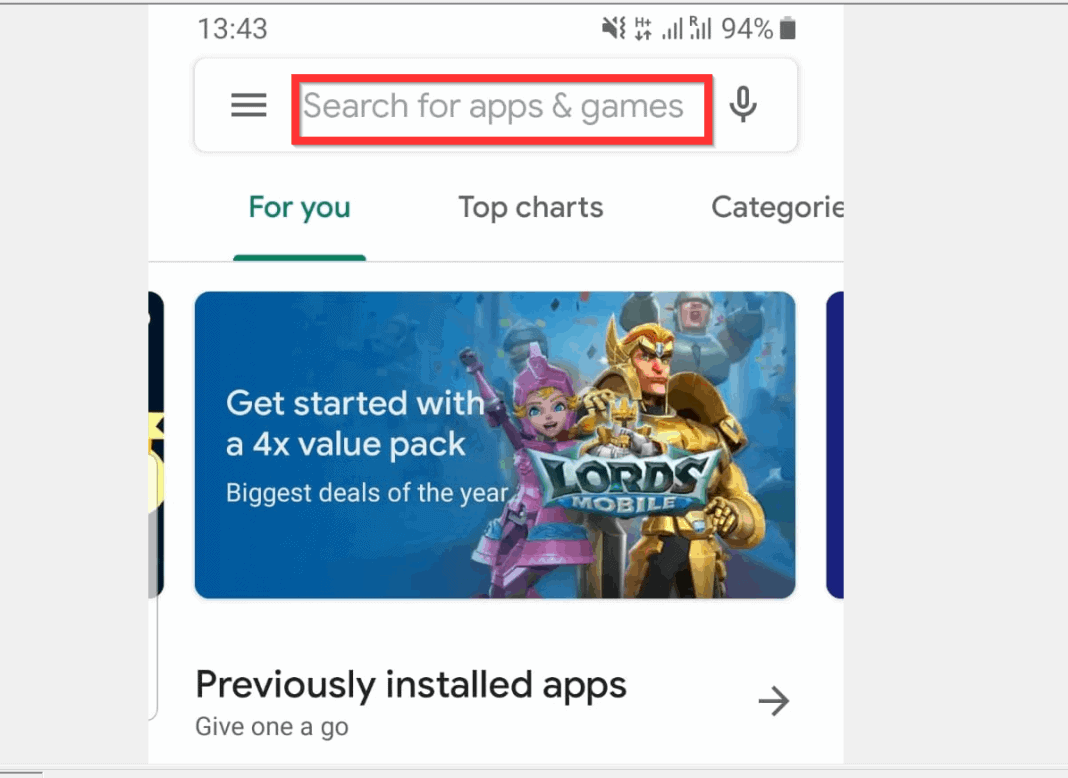The image shows a detailed close-up screenshot of a mobile device screen with a user interface typically seen in the Google Play Store. The time displayed is 13:43, indicated with a gray header at the top of the screen. The status bar includes several icons: signal indicators, a 94% battery level, an alarm icon turned off, and a few other unidentifiable icons.

Below the status bar, there's a hamburger menu icon followed by a search bar with the placeholder text "search for apps and games," highlighted by a red rectangle. To the right of the search bar is a microphone icon. This entire area is enclosed within a thin outlined rectangle that has a drop shadow effect.

Under the search bar are three navigation options: "For you," "Top charts," and "Categories." The "For you" tab is selected, evidenced by the green text and an underline bar.

Partially visible beneath this menu are two truncated rectangular thumbnails of app suggestions. The observable part of the left thumbnail reveals the game "Lords Mobile," featuring an illustration of a character in armor and a girl, possibly in armor or wearing a pink dress, standing to the left with her hand raised. There are also promotional texts like "Get started pack with 4x value pack, biggest deals of the year."

Further down, there's a text prompt that reads "Previously installed apps, give one a go," with an arrow pointing to the right. The arrangement and design elements suggest a promotional or suggestion section within the app interface.